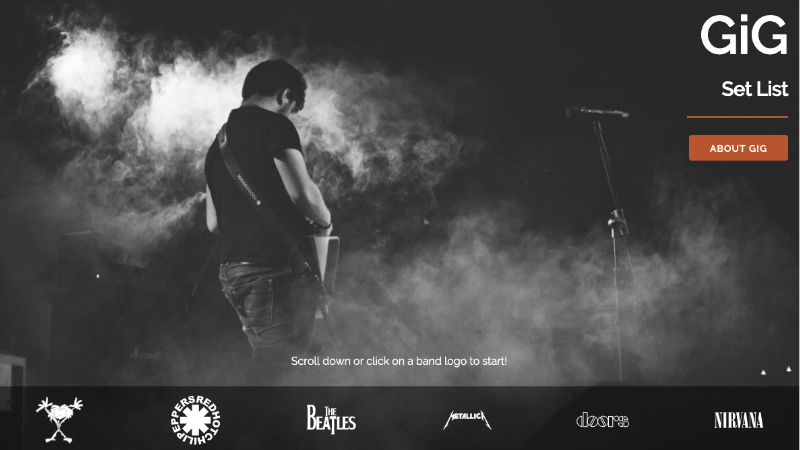A musician, captured mid-performance, is seen playing an instrument with their back to the camera, suggesting an intense moment of concentration. They are oriented towards the upper right-hand side of the image. The musician is dressed casually in a black short-sleeve t-shirt and jeans, with black hair visible. The instrument is secured with a strap that crosses their shoulder. To the right, a microphone stands ready, hinting at a live performance. In the background, the words "G.I.G." and "set list" are prominently displayed on the upper right corner, with an “about G.I.G." button visible behind the musician. Adding to the atmosphere, a smoky haze envelops the scene, intensifying the live performance vibe. To the left of the musician, an amplifier sits subtly in the background. A black bar runs along the bottom of the image listing renowned bands: Red Hot Chili Peppers, Beatles, Metallica, Doors, and Nirvana.